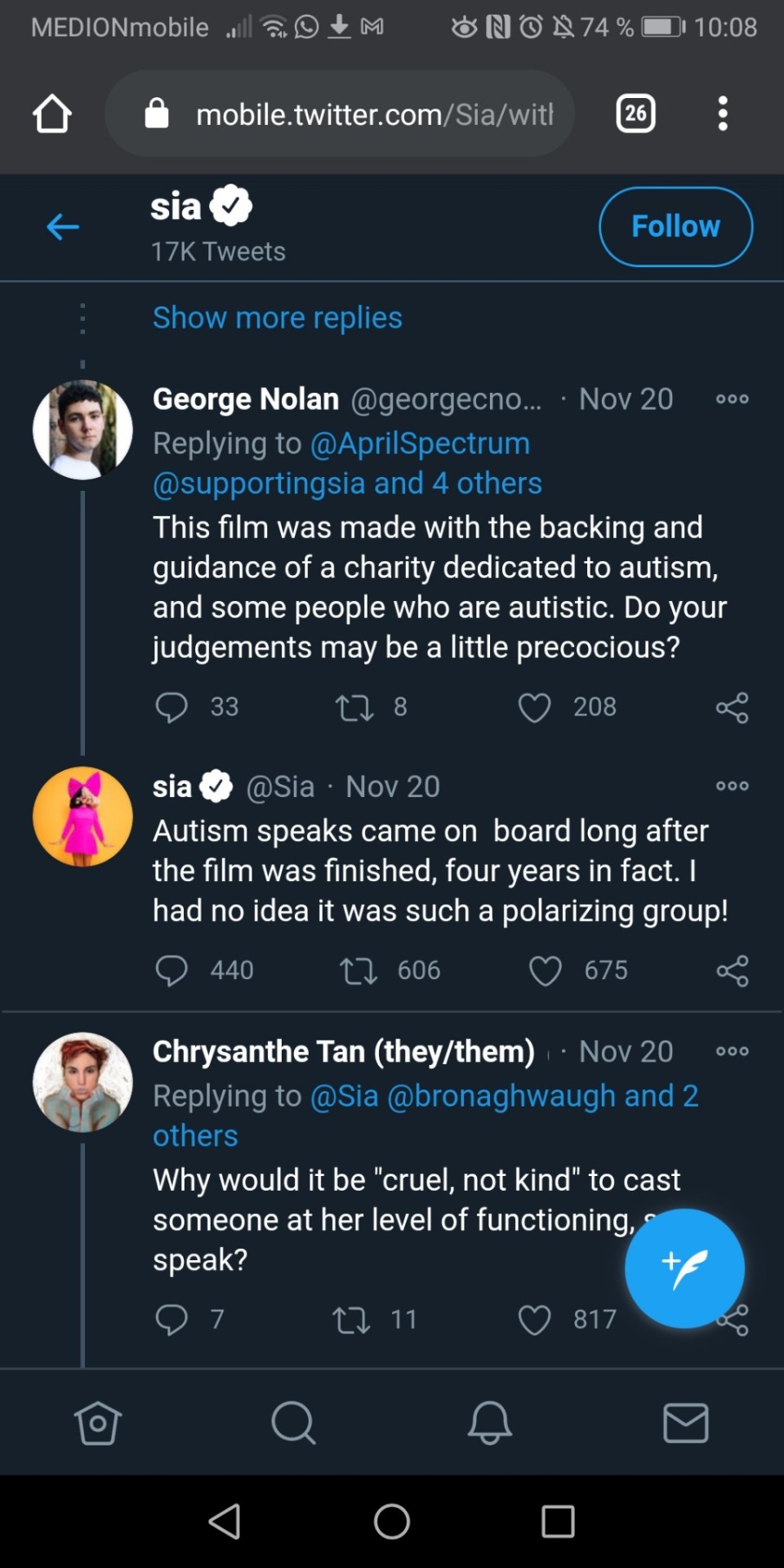This is a detailed screenshot of a Twitter page featuring a dark blue background. At the top, white text prominently displays the handle "CIA" accompanied by a white checkmark. Below it, in gray text, the number "17K Tweets" is shown. On the left side of the page, there's a blue back arrow, while to the right, a pill-shaped blue "Follow" button with a blue outline and text is visible. Below this, a blue link labeled "Show more replies" can be found. Underneath that, there is a tweet by George Nolan. His handle, "@GeorgeCNolan," is displayed in white, followed by an ellipsis. The tweet is a reply to "@AprilSpectrum" and "@supportingCIA and 4 others," with these handles shown in blue text. The content of the tweet states, "This film was made with the backing and guidance of a charity dedicated to autism, and some people who are autistic. Your judgments may be a little precocious."